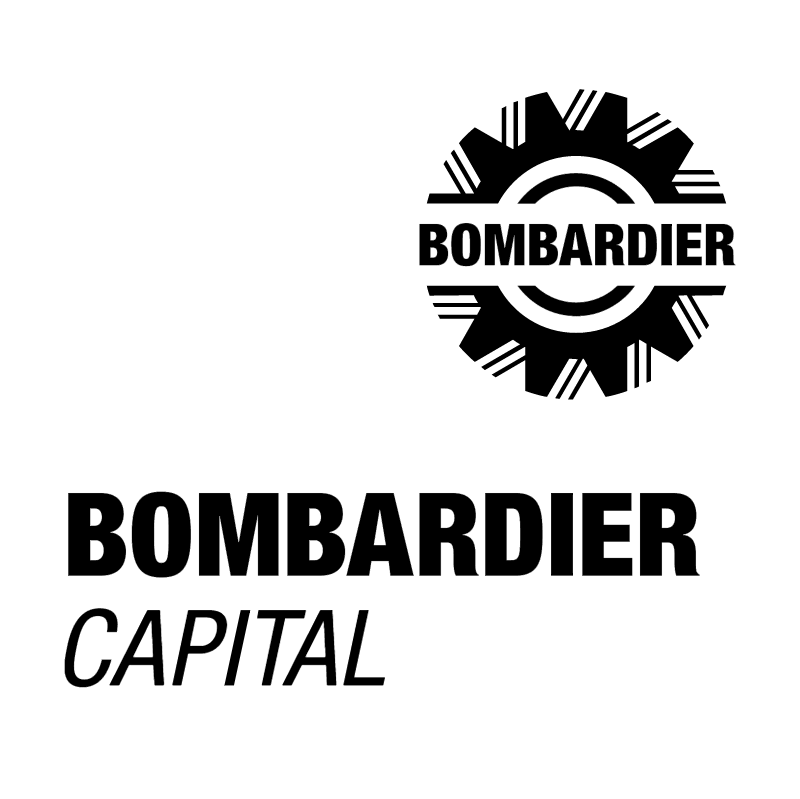The image features a black and white logo situated in the upper right corner on a pure white background. The logo consists of a circular, gear-like symbol with black rays extending around its perimeter. Within this gear-like symbol, the word "BOMBARDIER" is prominently displayed in bold, black, all-capital letters, cutting through the center of the circle. Aligned to the lower left of the image are two lines of text. The first line reads "BOMBARDIER" in bolded, black, all-capital letters. Directly below it, the second line reads "CAPITAL," also in black, all-capital letters, but thinner and italicized. Both lines are left-justified, harmonizing with the overall monochromatic and structured design of the logo.